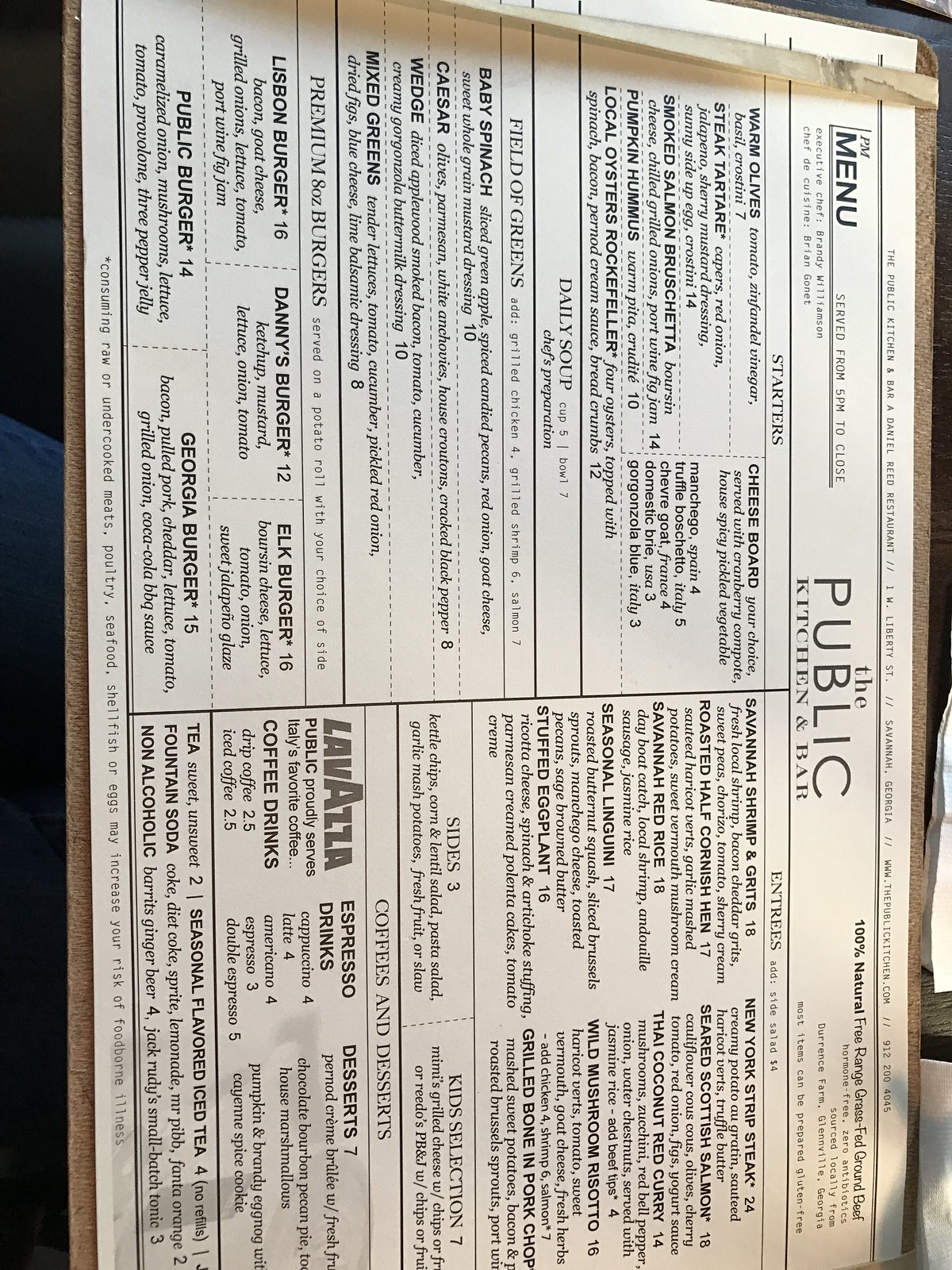The image showcases a large menu printed on white paper with black text, oriented sideways with a quarter turn to the right. At the very top, the menu prominently displays "The Public Kitchen and Bar" followed by the heading "Menu" in bold black ink. Below this, the menu is sectioned into various categories: "Starters" listing appetizers, starting with the "Daily Soup." Next is a section titled "Field of Greens" featuring an assortment of salads. Further down, there is a selection of burgers. A black line bisects the menu, leading to the other side, which details entrees that include various seafood, steak, and vegetarian/vegan options. At the bottom of this side, the menu lists coffee drinks, espresso drinks, and desserts, followed by iced tea and non-alcoholic drink options. The menu rests on a light brown wooden table, adding a rustic touch to the overall presentation.